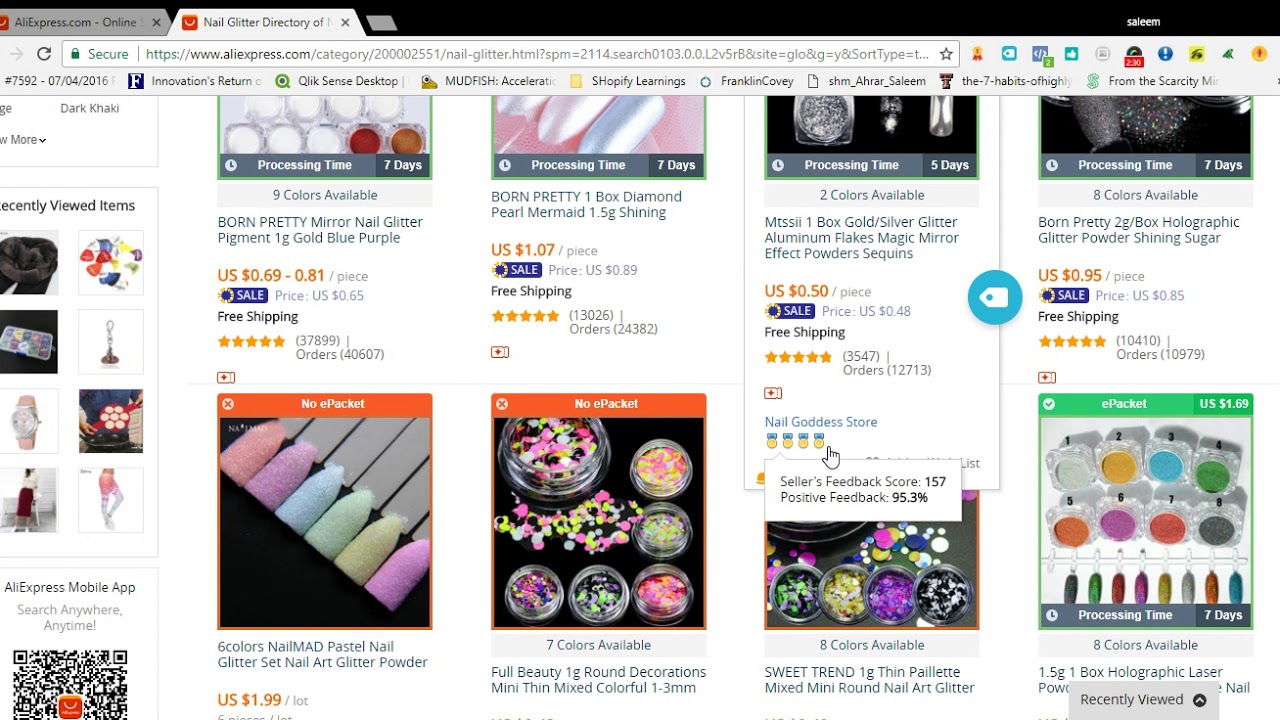This image is a detailed screenshot of a desktop or laptop displaying a web browser with a dark theme, focused on the website aliexpress.com. The page has a bright white background, creating a stark contrast with the dark-themed browser. There are two visible tabs: the active tab reads "Nail Glitter Directory of," while the adjacent tab is labeled "aliexpress.com." 

On the active tab, the webpage showcases a variety of fingernail decoration products arranged in a grid. Each product is presented with a square thumbnail image, followed by the product name, price, and shipping information. The user's white cursor, shaped like a hand with an extended finger, is shown hovering over the feedback score of a particular seller named "Nail Glitter Store."

The user has clicked on one of the products, causing the feedback score details to expand in a popup. This popup reveals the seller's feedback score of 157 and a positive feedback rate of 95.3%. The cursor specifically highlights four decorative medals associated with the seller. The intent of the screenshot appears to be to document this specific seller's feedback score and reputation metrics.